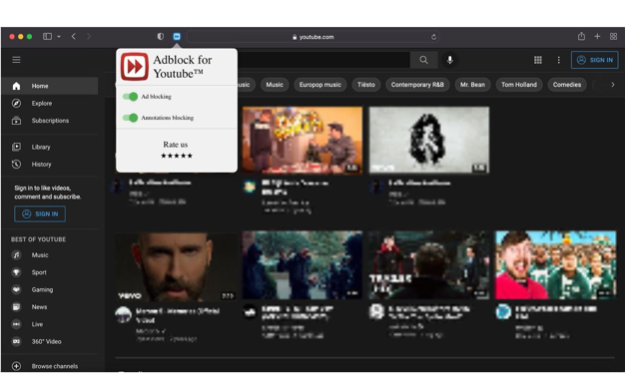The image depicts a screenshot of a YouTube webpage, primarily showcasing a music video section as indicated by the presence of various video thumbnails and the mention of "Vevo," a popular music video network. The URL at the top confirms that it is, indeed, YouTube.com. An 'Add Block for YouTube' extension interface is prominent in the image, having been activated by clicking a small icon at the top of the browser, which expanded into a larger overlay. This overlay includes several options: 'Add Block for YouTube,' 'Add Making,' 'Annotation Making' (though the text is partially obscured), and a 'Rate Us' section featuring five-clickable black stars for user ratings.

The YouTube page itself displays a series of video thumbnails organized in two rows. The top row consists of three clickable video thumbnails with images and the bottom row has four, each thumbnail accompanied by detailed information about the video's length and content description. The entire layout and content give the impression of a typical YouTube browsing experience focused on music videos, enhanced by the additional overlay interface.